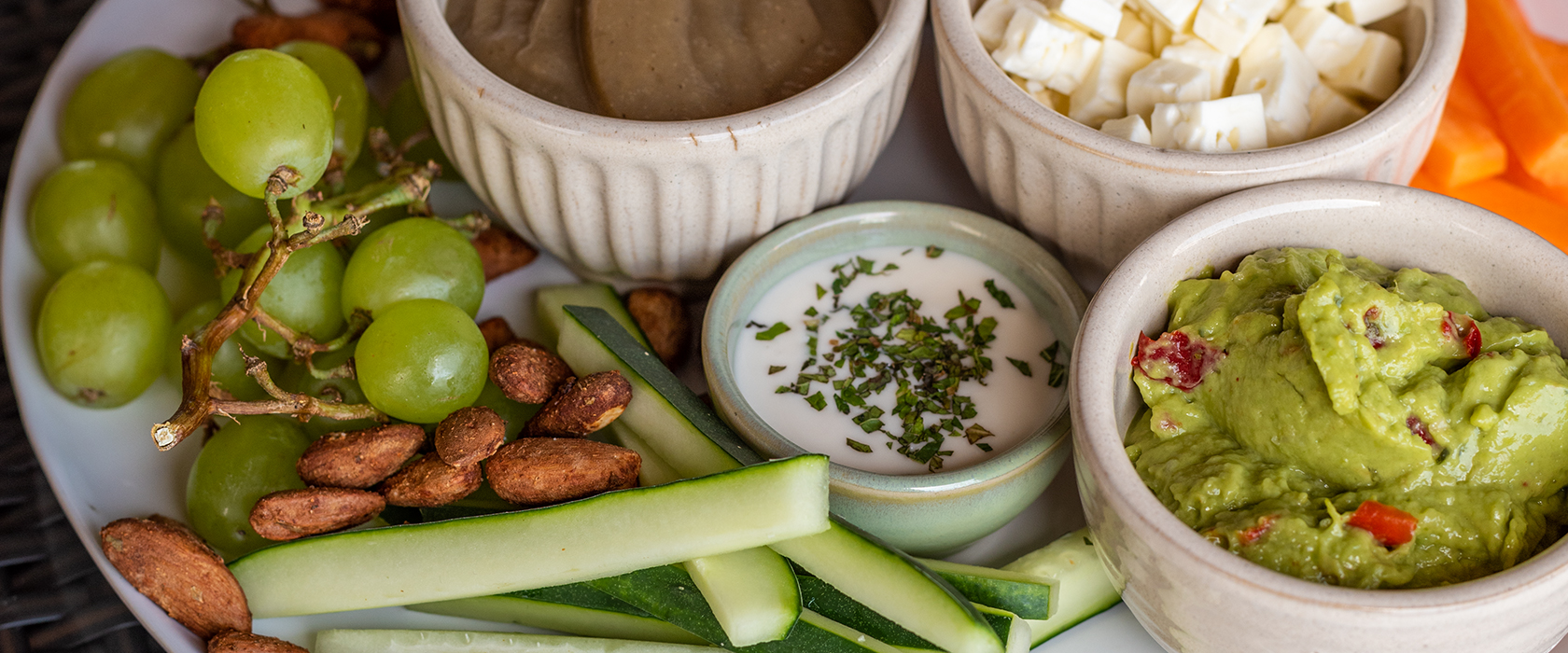A white plate brimming with an assorted array of foods is visually enticing. On the left side, clusters of green grapes, still on the vine, rest alongside a handful of mixed nuts, possibly peanuts, cashews, or almonds. Below them lie neatly cut sticks of cucumber. Towards the upper portion of the plate and slightly to the right, three white ceramic bowls are positioned. The center bowl contains a creamy white dip speckled with green herbs, likely a type of ranch dressing. To its immediate right, a bowl holds guacamole mixed with vivid red pimentos. The bowl to the far right contains white blocks of cheese or tofu. Additionally, a smaller blue bowl also features on the plate, holding what could be a brown sauce or perhaps cooked apples. Scattered around the edges of the plate, the ends of fresh carrots are visible. The entire arrangement is set atop a brown mat, enhancing the rustic appeal of this diverse and inviting spread.